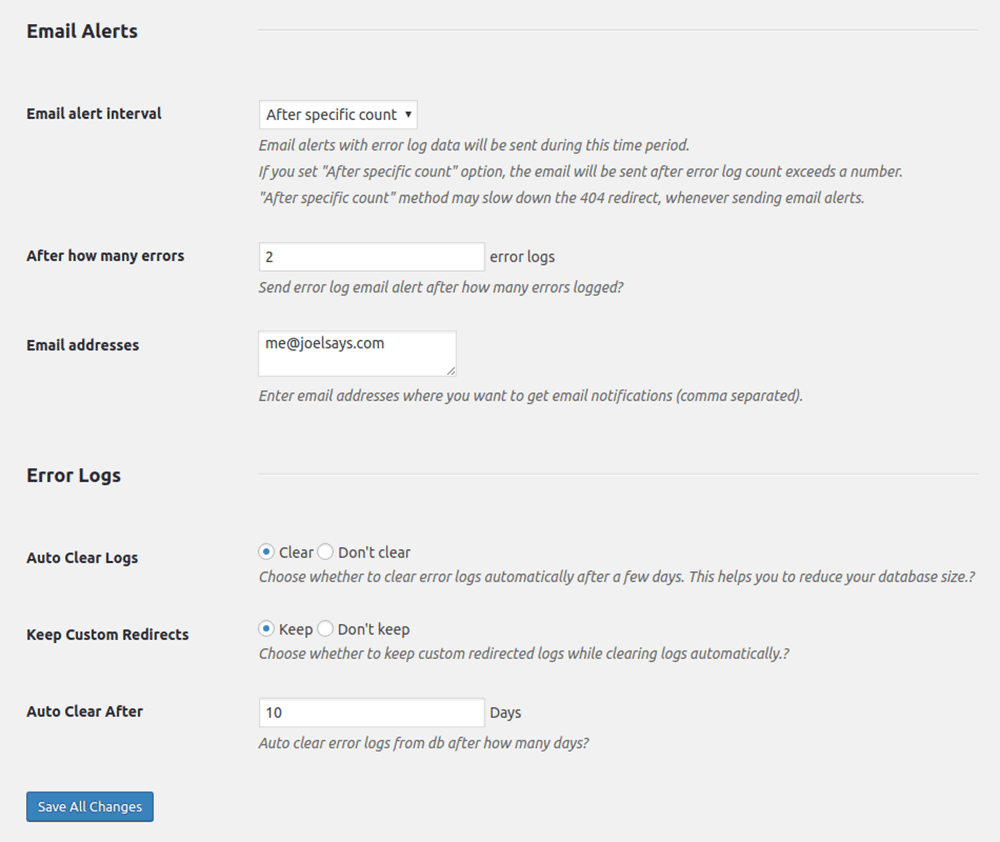The image captures a screenshot of a web interface on a computer, specifically a settings page for email alerts. The background is a very light blue-gray color. 

At the top left, the title "Email Alerts" is displayed in black font. On the left-hand side of the screenshot, there are various sections and paragraphs that outline different settings options.

Highlighted prominently in dark black font is a section labeled "Email Interval After How Many Errors." Within this section, it specifies a threshold of two error logins before sending an alert. The designated email address for these alerts is "me@joelsays.com."

At the very bottom of the interface, there is a button labeled "Save All Changes," indicating the option to save any adjustments made in the settings.

Additional settings include options for managing error logs. There is a setting for automatically clearing logs, which is marked as "Clear." Another setting labeled "Keep Custom Redirects" is marked as "Keep." The auto-clear logs feature is set to activate after 10 days.

Overall, the interface is clean and straightforward, providing configurable options for email alerts and error log management.